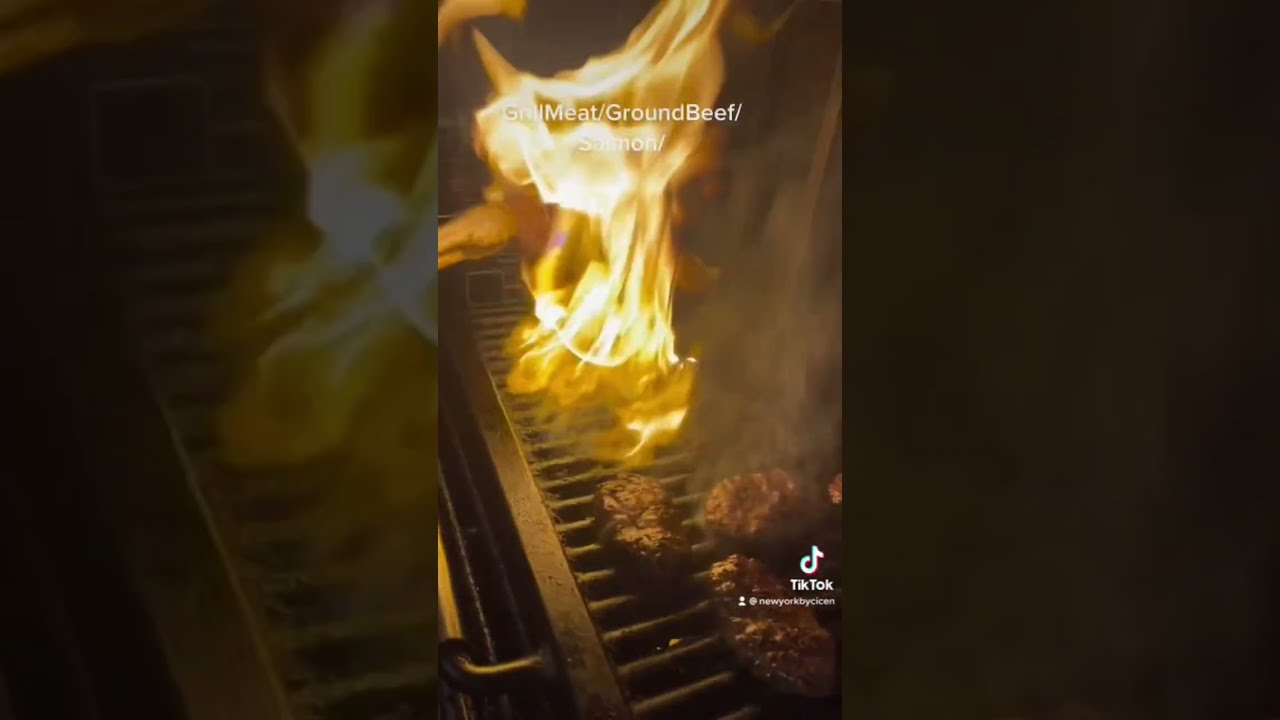In this image, a high flame erupts from a large black grill, with the fire reaching roughly a foot in height and transitioning from orange to white at its peak. The grill is predominantly black with a partially visible metallic handle, possibly with wooden elements. At the center of the grill, three to four patties of ground beef or steak are cooking, surrounded by substantial smoke. Overlaid in white text above the flame are the words "grill meat" and "ground beef," with a mention of "salmon" on the next line. A pair of tongs is seen flipping additional meat in the background, to the left of the large fire. The lower right corner of the image displays a white TikTok logo, indicating that this is a screenshot from a TikTok video. The image is bordered on the left and right by darker, fuzzier versions of the same scene, highlighting the central fiery spectacle.